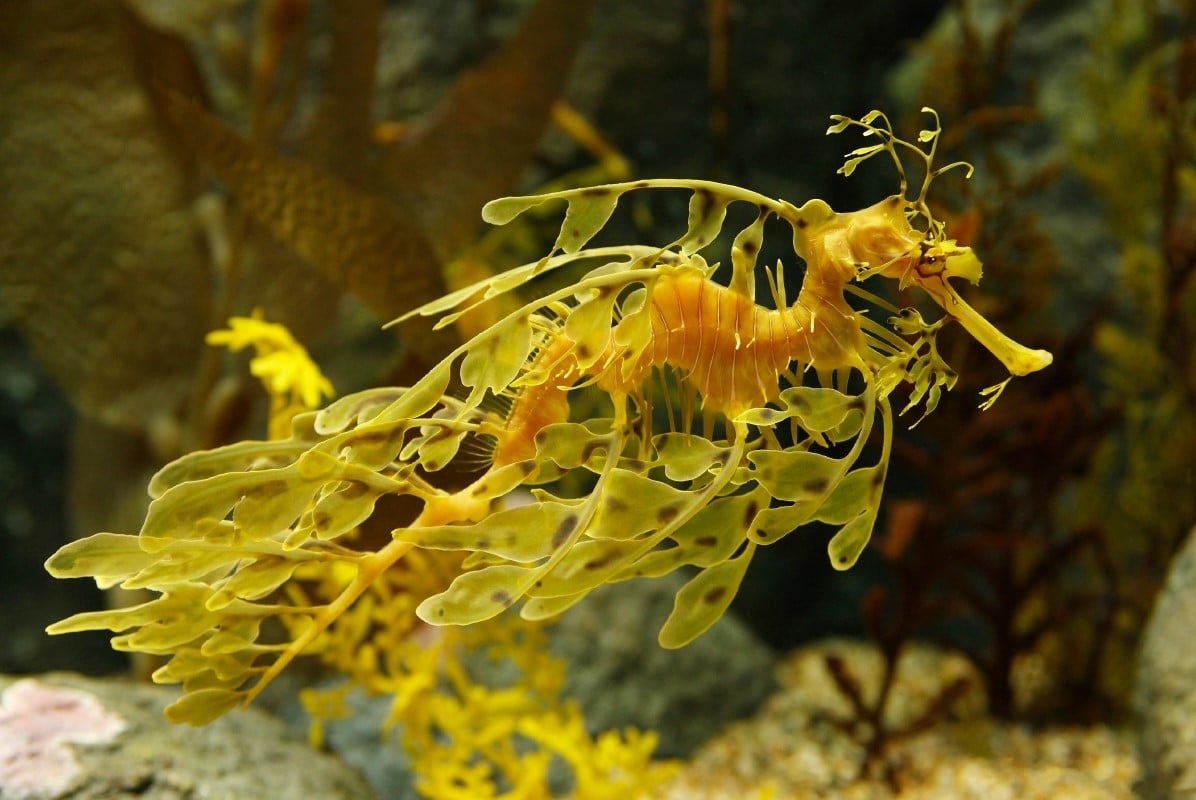This underwater photograph captures a bright yellow seahorse adorned with vine-like tendrils that resemble seaweed or kelp, giving it a camouflaged appearance. The seahorse's traditional, yet slightly misshapen head features an elongated, trumpet-like nose and spindly antennae. The body of the seahorse, which appears wave-like with visible vertebrae, is lined with greenish tendrils speckled with brown spots, enhancing its natural disguise. The background reveals a vibrant underwater scene with multicolored rocks and intricate coral structures, adding depth to this mesmerizing marine tableau.